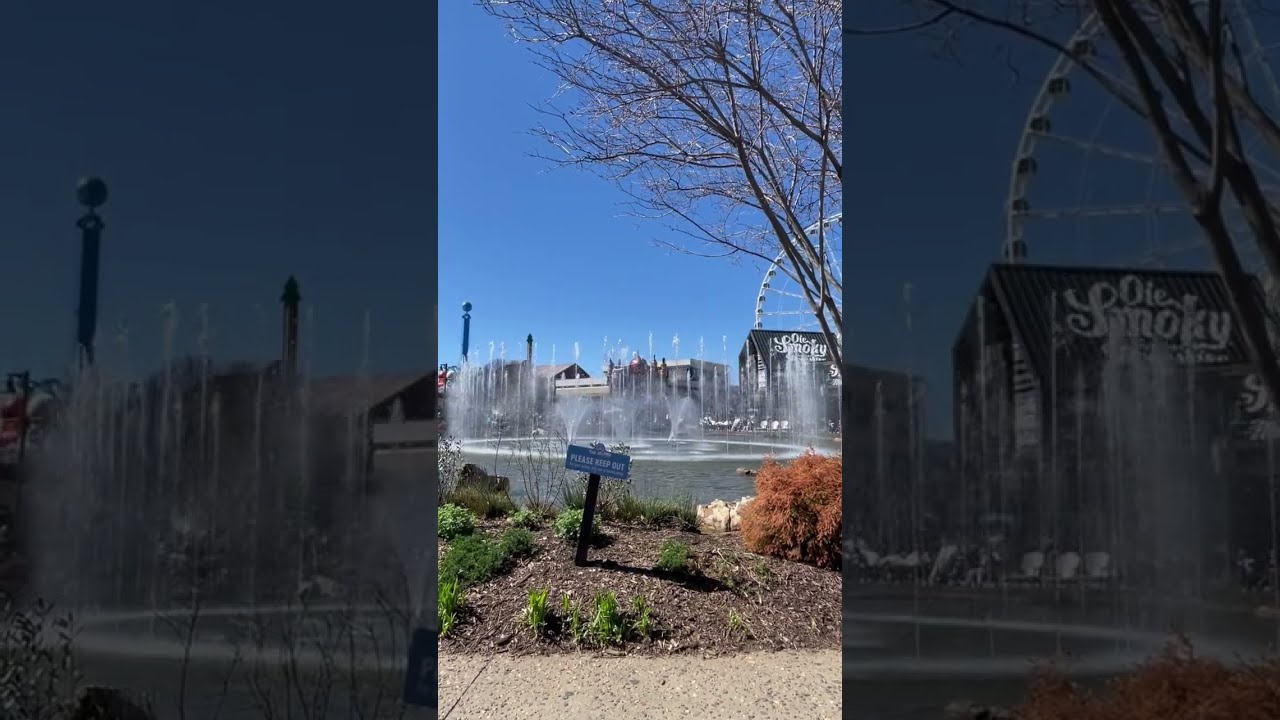This image captures a vibrant park scene with a clear, blue sky overhead. At the center of the photograph is a circular water body featuring an ornate fountain. The fountain has multiple spouts arranged in a circle, shooting water upwards in arches, with additional spouts in the center creating a dynamic display. Surrounding the pool, on the near edge, is a patch of soil and grass where a prominent blue sign reading "Please Keep Out" is staked into the ground. To the right, the skeletal branches of a dry tree frame the scene, while in the distance, tall buildings and parts of a Ferris wheel are visible, adding urban context to the natural setting. The ground features various colors, including the gray of a concrete path, the brown of the dirt, and the green of surrounding shrubbery. The overall composition suggests a casual snapshot taken during a leisurely walk in what appears to be a public park.